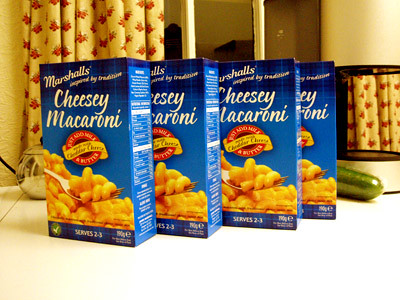This photograph evokes a nostalgic 1950s ambiance, featuring four meticulously arranged blue boxes of Marshall's Cheesy Macaroni on a white kitchen counter. Each box displays an appetizing image of macaroni on a fork, set against a backdrop of a yellow curtain adorned with red fruit patterns and green leaves. The window sill, painted in light yellow wood, complements the lighter yellow wall. Additional details on the boxes include a red circle with promotional information, a yellow banner, and a blue banner likely containing nutritional information. A green cucumber, or possibly a green-handled utensil, is partially visible behind the last box, adding a touch of realistic kitchen clutter to the scene.